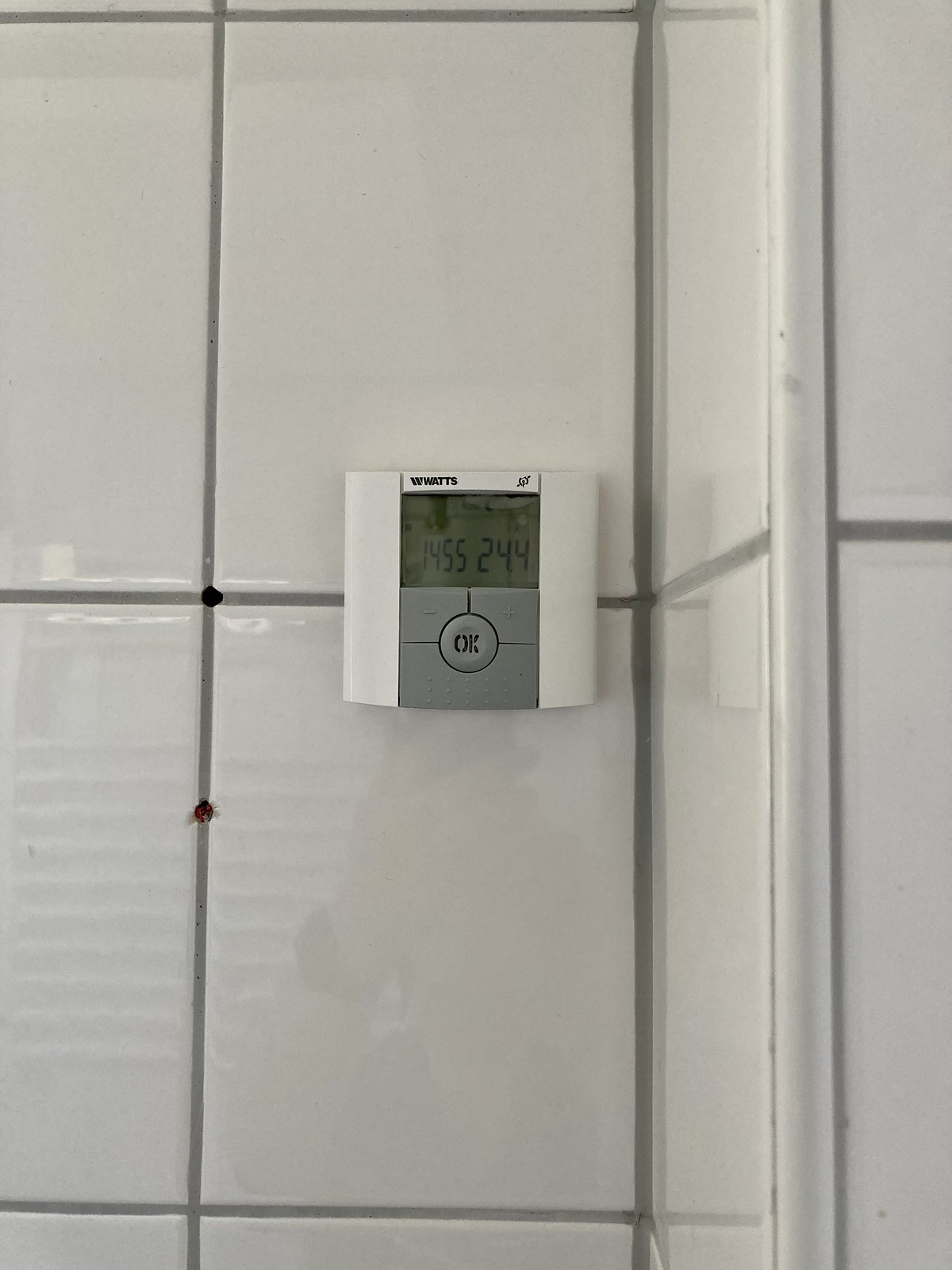This image features a close-up view of a digital device mounted on a wall, possibly a thermostat or a similar control device. The device is located in a corner of a tiled wall, which appears to be a shower area based on the arrangement and type of tiles. The wall is covered with white tiles separated by gray grout lines, and the corner reveals tiles on two intersecting walls.

The device is white with a digital display in the center showing the numbers "1455244." At the top of the device, the brand name "Watts" can be seen. Beneath the digital display is a gray "OK" button. The image's perspective highlights the device's flat positioning against the wall, with visible portions of about one and a half tiles on both the left and right sides. The corner shows a border running vertically through the tiles, adding a straight, clean line to the design.